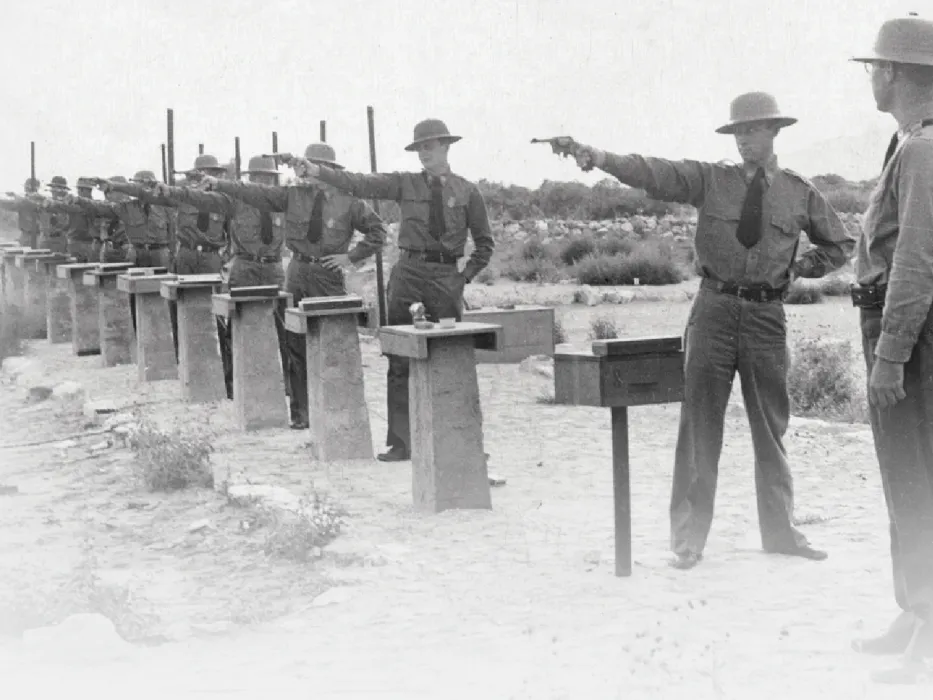This black-and-white photo presents a historical scene of a military firing range exercise. A line of approximately 15 soldiers stands in formation, each positioned by a concrete pedestal with a tray on top to hold their belongings. These men are in uniform, wearing hats with brims, long-sleeve button-up shirts, short ties, belts, and trousers. With their right arms outstretched, each soldier grips a firearm, pointing it forward in unison. The scene is set against an outdoor backdrop with a clear sky, distant trees, and a rocky, dusty field. On the far right side of the image, an officer or instructor, dressed similarly but without a firearm, observes the soldiers, indicating his supervisory role. The overall scene captures a moment of disciplined military practice in a stark, open environment.